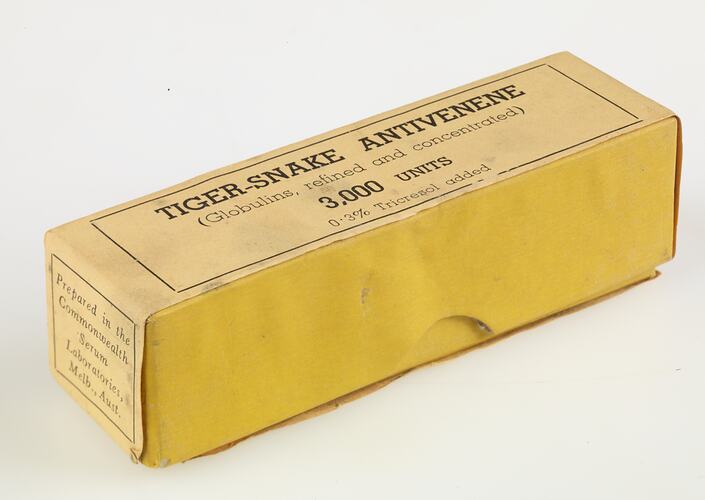The image features an old-looking, rectangular carton with a flip-open design, set against a light gray or off-white background. The box, in a worn yellowish-orange color, is diagonally positioned from the bottom-left to the upper-right. Bold black text on the top of the box reads "Tiger Snake Anti-Venene," indicating it is a type of anti-venom medication. Below this, it states "Globulins Refined and Concentrated, 3,000 units" and "0.3% Trichronyl Added." Additionally, the side of the box bears the inscription "Prepared in the Commonwealth Serum Laboratories, Melbourne, Australia," though the text is partially obscured by the angle of the photo.